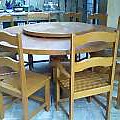The image, which is a very small, square thumbnail, depicts a round wooden table in what appears to be a kitchen or a dining room area. The table features a Lazy Susan, a smaller round piece of wood in its center, used for placing items that can be spun around. Surrounding the table are several wooden chairs; two of them, clearly visible at the front, are light brown, with slatted backs and no armrests. One chair in the front right is distinguished by a cushion, suggesting it is either upholstered or has a separate cushion for added comfort. The table and chairs are situated on a floor covered by a rug with white, tan, gray, and black patterns. In the background, the white walls with brown trim complement a kitchen setting, enhanced by the presence of what seems to be a fish tank on a counter. Despite the image's tiny size and lack of detail, these elements suggest a cozy, well-decorated kitchen or dining area meant for both practicality and comfort.